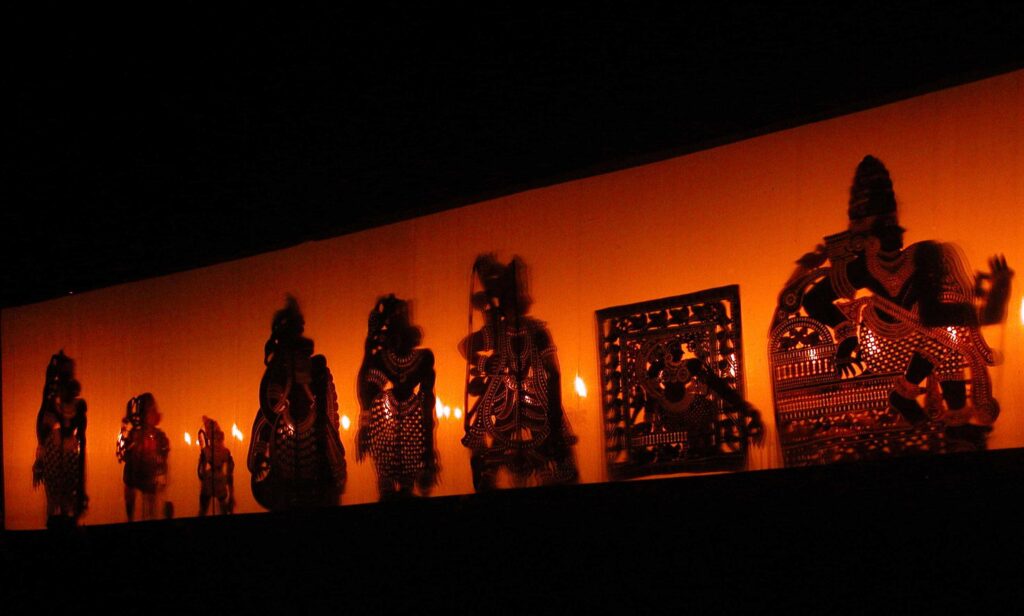The image depicts a dimly-lit indoor setting with a vibrant orange backdrop. The ceiling and floor are both shrouded in darkness, obscuring any details. The focal point of the image is a horizontal, rectangular section illuminated by a golden glow, reminiscent of a theater stage or curtain. Scattered across this orange backdrop are various metallic sculptures, possibly made of gold or bronze, though the lighting casts deep shadows that make it difficult to discern their true color and finer details. 

On the left side, there are three smaller statues that appear to be children, while towards the center and right, three much larger statues stand, resembling adult figures. Interspersed among these statues, second from the right, is a distinctive square adorned with ornate metalwork. To the far right, a particularly large and detailed figure seems to be intricately designed, possibly holding something resembling a chest. Reflective lights highlight portions of these statues, further enhancing the mysterious and shadowy ambiance of the scene.